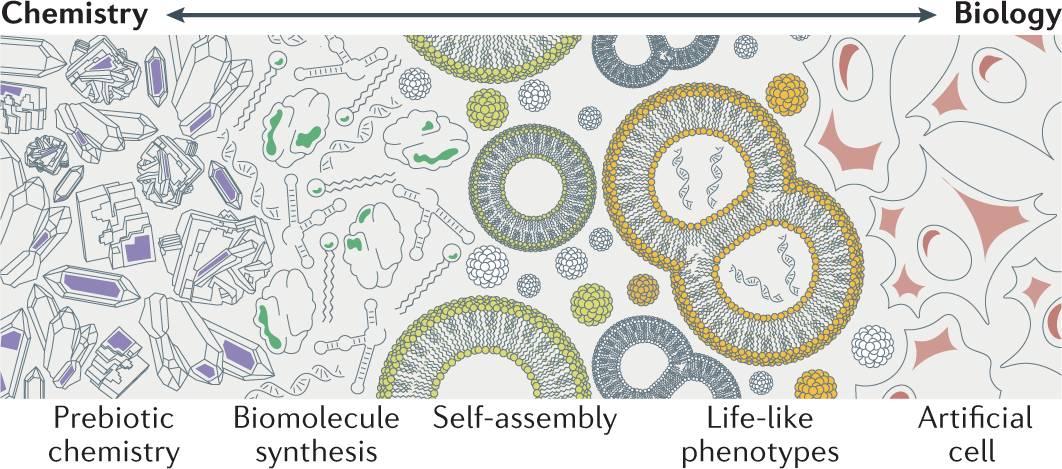This detailed and colorful graphic serves as a stylized rendering, possibly for a medical journal poster depicting the transition from chemistry to biology. At the top, the word "Chemistry" is prominently displayed on the left, while "Biology" is on the right, connected by a double-headed arrow. Below this, an intricate line drawing illustrates various stages of this transition. The illustration is more densely packed on the chemistry side (left), with black and white figures accented by purple regions. As you move towards the center, the drawing transitions to green-toned shapes that are more organic and rounded. The central area features more elaborate decorations in gold and orange colors, representing intermediate molecular structures. On the far right, symbolizing biology, the figures become more dispersed and simplified, utilizing a pinkish color palette.

Underneath this drawing, a sequence of terms runs from left to right, correlating with the illustrations above them: "Prebiotic Chemistry," "Biomolecule Synthesis," "Self-Assembly," "Lifelike Phenotypes," and "Artificial Cell." Each term is visually represented by different shapes and colors that transition consistently from purple through green, gold, orange, to pink. These elements collectively illustrate the shift from chemical compounds to biological structures, encapsulating complex scientific concepts in an accessible and visually engaging manner.